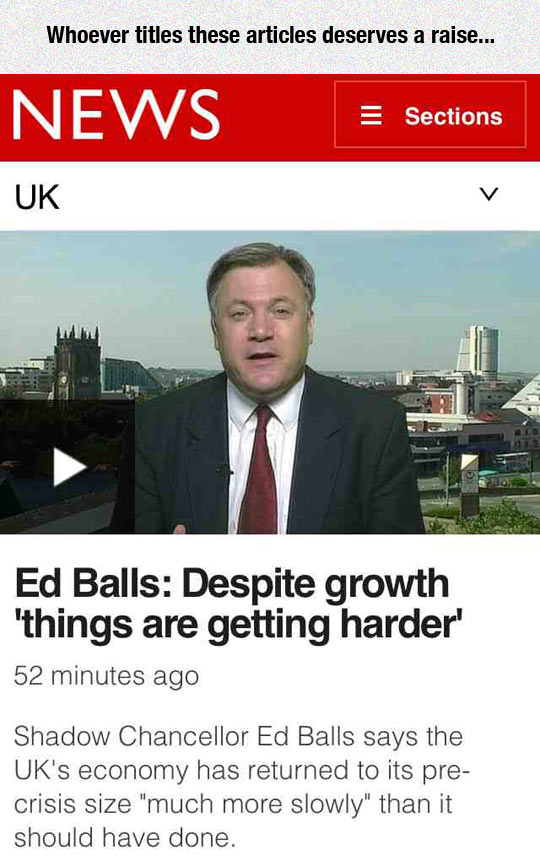The image depicts the homepage of a news website, characterized by its clean, modern layout. At the very top, a gray banner prominently features a statement in white text: "Whoever titles these articles deserves a raise." Below this banner, a red headline bar displays the word "News" in bold white letters, which is flanked by a clickable section on the right labeled "Sections."

In the main content area, there is a feature article marked as originating from the UK. The focal point of this article is a photograph of an elderly man, dressed in a suit and tie, sitting against the backdrop of a cityscape. Overlaying the photo is a play button, suggesting the availability of a video clip. The headline associated with the image reads: "Ed Balls: Despite growth, things are getting harder." This article was posted 52 minutes ago.

The article provides a brief summary in a light blue-gray font, stating: "Shadow Counselor Ed Balls says the UK's economy has returned to its pre-crisis size much more slowly than it should have been." This concise description encapsulates the current economic challenges as highlighted by Ed Balls.

The overall composition of the image suggests a professional, user-friendly news platform dedicated to providing timely and incisive reports.